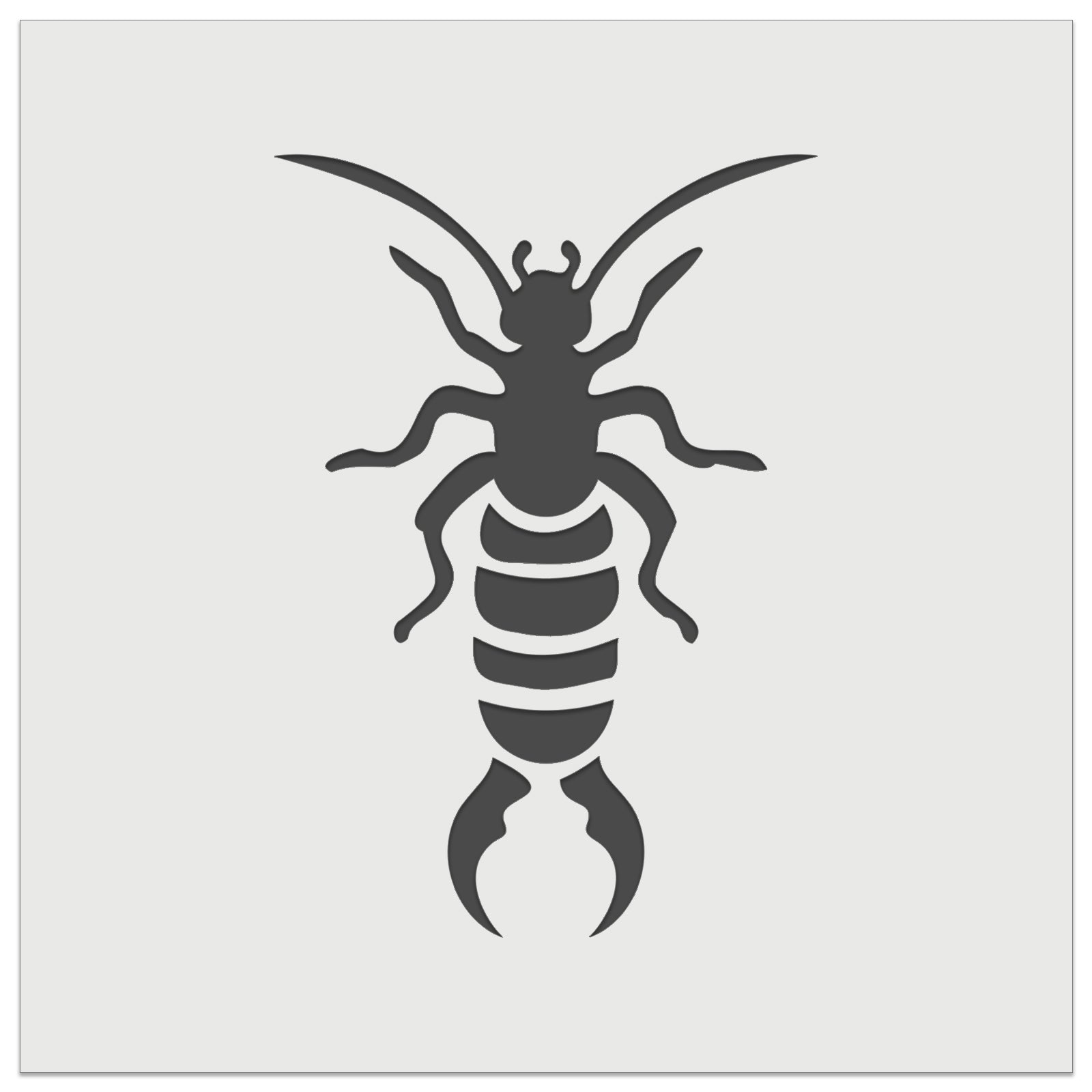The image depicts a detailed, digitally-created design of an insect. The artwork is not hand-drawn but appears to be crafted using a digital program, showcasing intricate details that suggest the insect belongs to a recognizable species, though the exact type is undefined. The insect sports six legs, affirming its classification, and features a notably elongated hind quarter, nearly as long as its body. The hind quarter terminates in two pincer-like structures, likely intended for intimidation or defense, creating the illusion of a second head to deter predators. This clever adaptation helps mislead threats into attacking the false head instead of the actual one. The entire piece is rendered in black and white, emphasizing the stark and simplistic beauty of the insect's form and proportions.